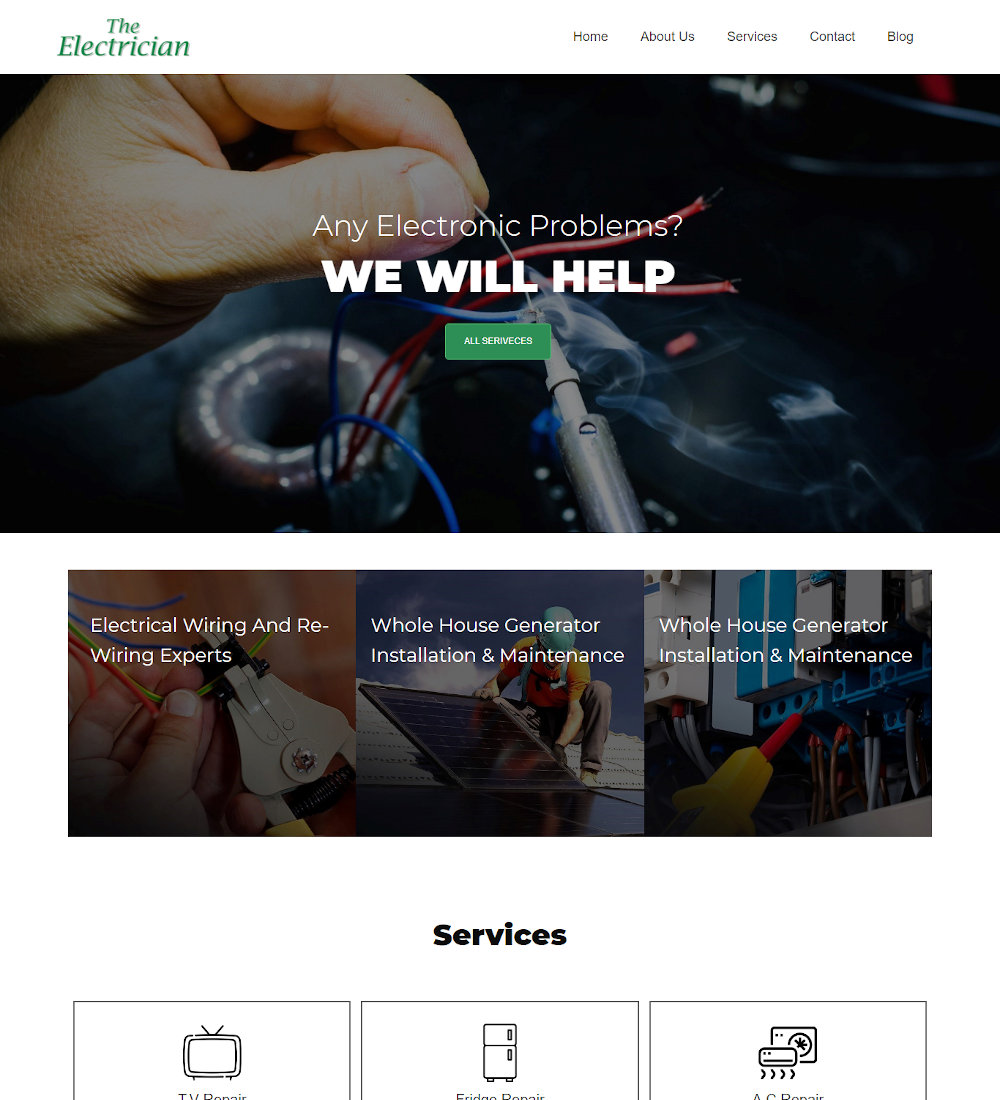Screenshot of "The Electrician" Website.

The screenshot features the homepage of a website titled "The Electrician," with the title prominently displayed in green letters at the top. To the right of the title, the website navigation menu includes the options: Home, About Us, Services, Contact, and Blog.

Central to the screenshot is a photograph depicting a person engaged in electrical work, accompanied by the text: "Any electronic problems? We will help. All services."

Below this, a list highlights the service offerings:
- Electrical Wiring and Rewiring Experts
- Whole House Generator Installation and Maintenance (repeated)
- TV Repair
- Fridge Repair
- AC Repair

The screenshot also includes three additional images. The first image shows a person working on a wiring project. The second captures an individual installing a solar panel on a roof. The third image displays an open electrical box with numerous wires visible.

At the bottom of the screenshot, there are drawings of a TV set, a refrigerator, and an air conditioning unit. The image does not contain any animals, plants, flowers, trees, automobiles, motorcycles, or bicycles.